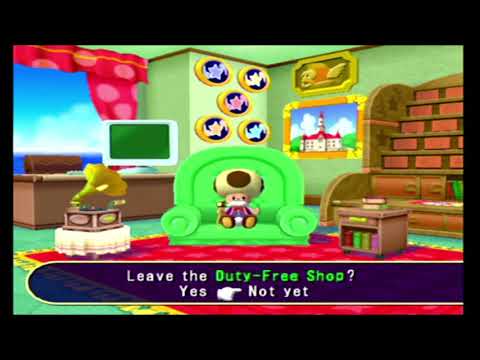This is a vibrant, color-rich scene from a Mario Party video game, featuring the character Toadsworth, who is easily recognizable by his cream-colored cap with brown spots and a little mustache. Toadsworth is comfortably seated in a bright lime green armchair. Surrounding him is a cozy, detailed setting that includes various elements: a red carpet underneath the chair, a brown stand, and an old-fashioned phonograph to his left. The background is adorned with red curtains, a picture window showcasing a blue sky and body of water, an array of shelves with books and red objects, and walls decorated with framed gold stars and a framed picture of one of the iconic Mario castles. On the right, there’s a small side table, more shelves, and a desk with a chair and another monitor. A text box spans the bottom of the screen, with a prompt in white and green text asking, “Leave the duty-free shop?” The options “Yes” and “Not yet” are presented, with a cursor currently pointing to “Not yet.” The black bands above and below frame the image, completing this colorful depiction of a scene filled with nostalgic and familiar Mario elements.